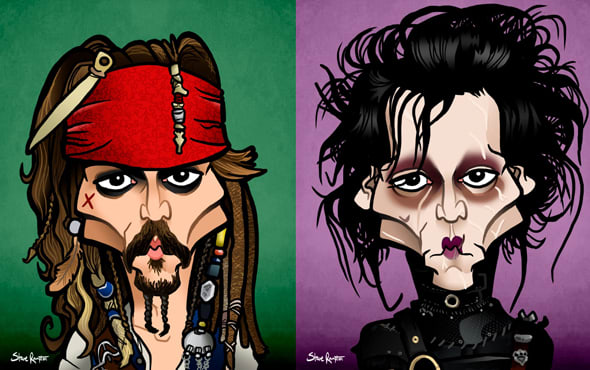The image showcases two detailed caricature drawings of characters portrayed by Johnny Depp in his movies. On the left, set against a green background, the character is dressed as a pirate, reminiscent of Captain Jack Sparrow. He wears a red bandana over his forehead, with long brown hair styled in dreadlocks and adorned with beads. His face features black eyes with red X mark below the right eye, eye makeup, and a mustache alongside a goatee tied into two braids that extend down to his neck. 

On the right, a character depicted against a moody purple background exudes a gothic vibe. Sporting wild jet black hair, he has pale skin with distinct purple-tinted lips and dramatic brown and purplish eye makeup. The character is dressed in a dominatrix-style black leather outfit accentuated with gold links. Additionally, there is a small, white initial located at the bottom left corner of the image, tying the two drawings together.